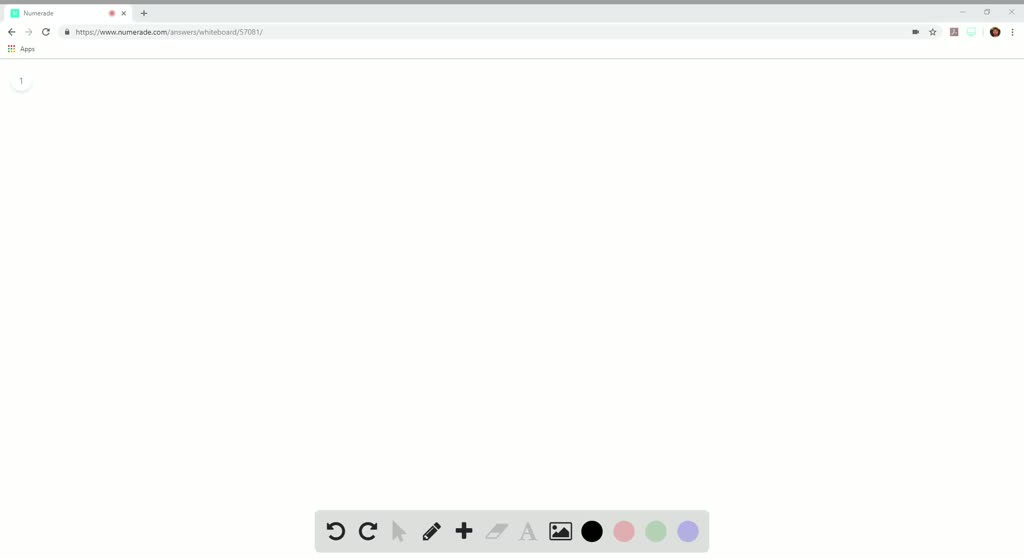This detailed descriptive caption provides a clear depiction of the screenshot:

---

The screenshot is very tiny, featuring a web browser with several elements. In the top left corner, there's a green logo followed by an indistinguishable word beginning with the letter "N" due to its small size. Beneath this, the URL bar displays a web address starting with "http://www." but the exact URL is unreadable because of its diminished clarity. Next to the URL bar, on the left, there is a left arrow and a refresh button, followed by three or four additional small icons. Below this row, the bookmark bar is visible with an "Apps" button.

The main portion of the webpage content area is entirely blank, except for a small circle in the top left corner containing the number "1". At the bottom of the screenshot, there is a toolbar with several icons: a circular arrow pointing left, a circular arrow pointing right, an arrow pointing to the top right, a pencil icon, a plus icon, an eraser icon, a text icon, and an image icon. Additionally, there are four color circles at the bottom: one black, one red, one green, and one purplish-blue.

---

This caption provides a comprehensive and detailed description suitable for understanding the intricate features of the screenshot.